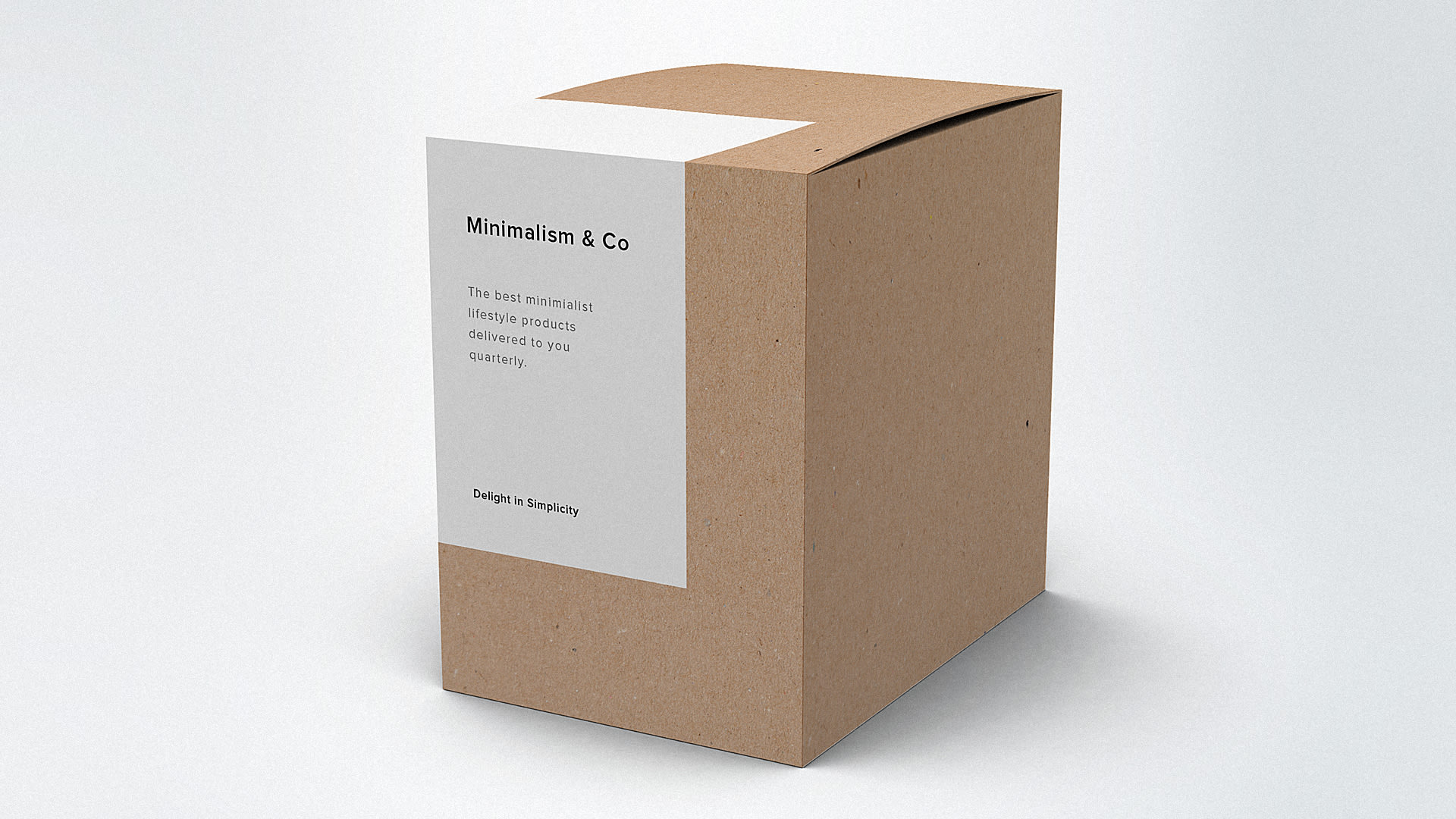The photograph features a plain, light brown cardboard box situated against a stark white background. The box prominently displays a white label that covers approximately two-thirds of its front panel and extends over the top flap. The label contains black text with a minimalist aesthetic, reading "Minimalism and Co" at the top. Below this title, the label states, "The best minimalist lifestyle products delivered to you quarterly," in smaller print. At the bottom of the label, the phrase "Delight in Simplicity" is visible. The box’s top flap is slightly ajar, revealing a darker shadowed interior. This subtle opening gives a sense of depth to the box. Additionally, a small, darker brown line is visible on the top right corner, indicating the box lid is slightly beveled upward. The light source in the image appears to be from the top left, casting a shadow to the right of the box, enhancing its three-dimensional appearance.